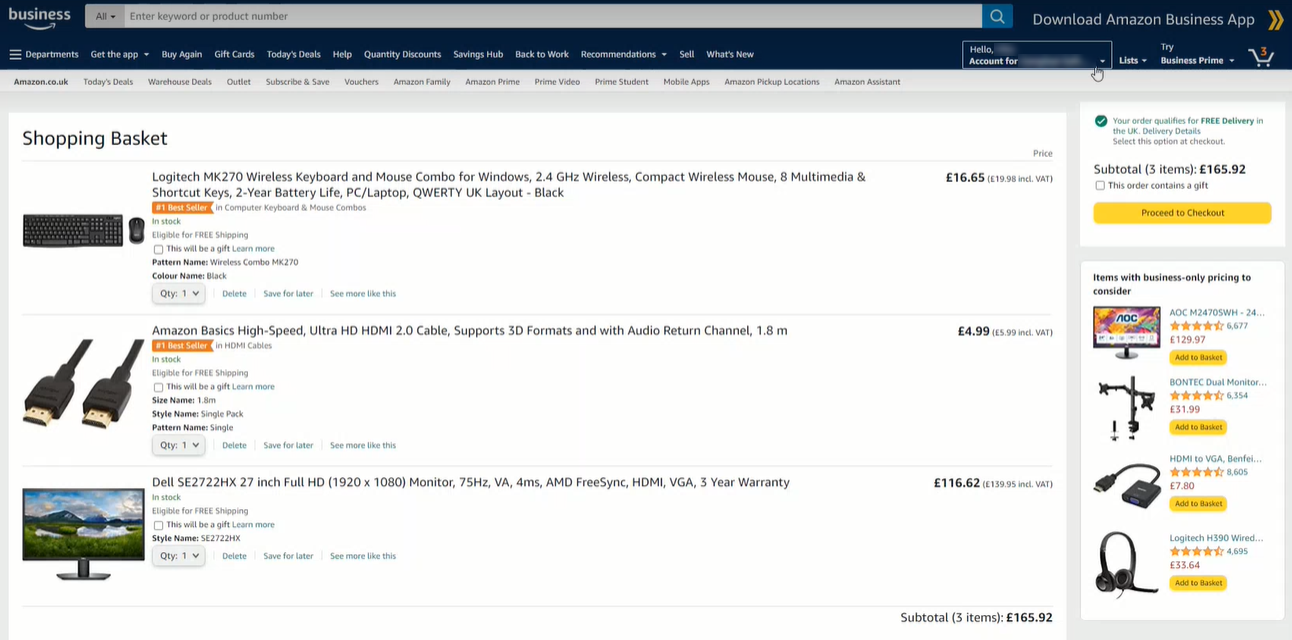This screenshot captures the Amazon Business webpage, presenting a busy and detail-oriented user interface. At the top center, the image features the "Amazon Business" logo, complete with the iconic Amazon smile. Prominently displayed underneath is a search bar with the placeholder text "Enter keyword or product number" and is currently set to search "All" categories. Adjacent to the search bar is a light blue search button, while the far-right side of the header includes a downloadable link for the Amazon Business app, indicated by two yellow chevrons pointing to the right.

Below the search bar, a navigation menu displays several key options: "Departments," "Get the App," "Buy Again," "Gift Cards," "Today's Deals," "Help," "Discounts," "Savings Hub," "Sell," "What's New," and additional links that are pixelated and slightly difficult to decipher. Further to the right, there's a "Hello" section for user profile management, including lists, a "Try Business Prime" invitation, and an Amazon cart icon mirroring the number of items, which is three in this instance.

Within the cart, identified as the "shopping basket," the items listed include: a Logitech Wireless Keyboard, an Amazon Basics High-Speed Ultra HD HDMI Cable, and a Dell 27-inch HD Monitor. To the right of the cart, suggestion widgets offer business-specific pricing on additional items: a monitor, a monitor stand, an HDMI to USB converter, and a headset, allowing for enhanced productivity and streamlined purchasing for business needs.